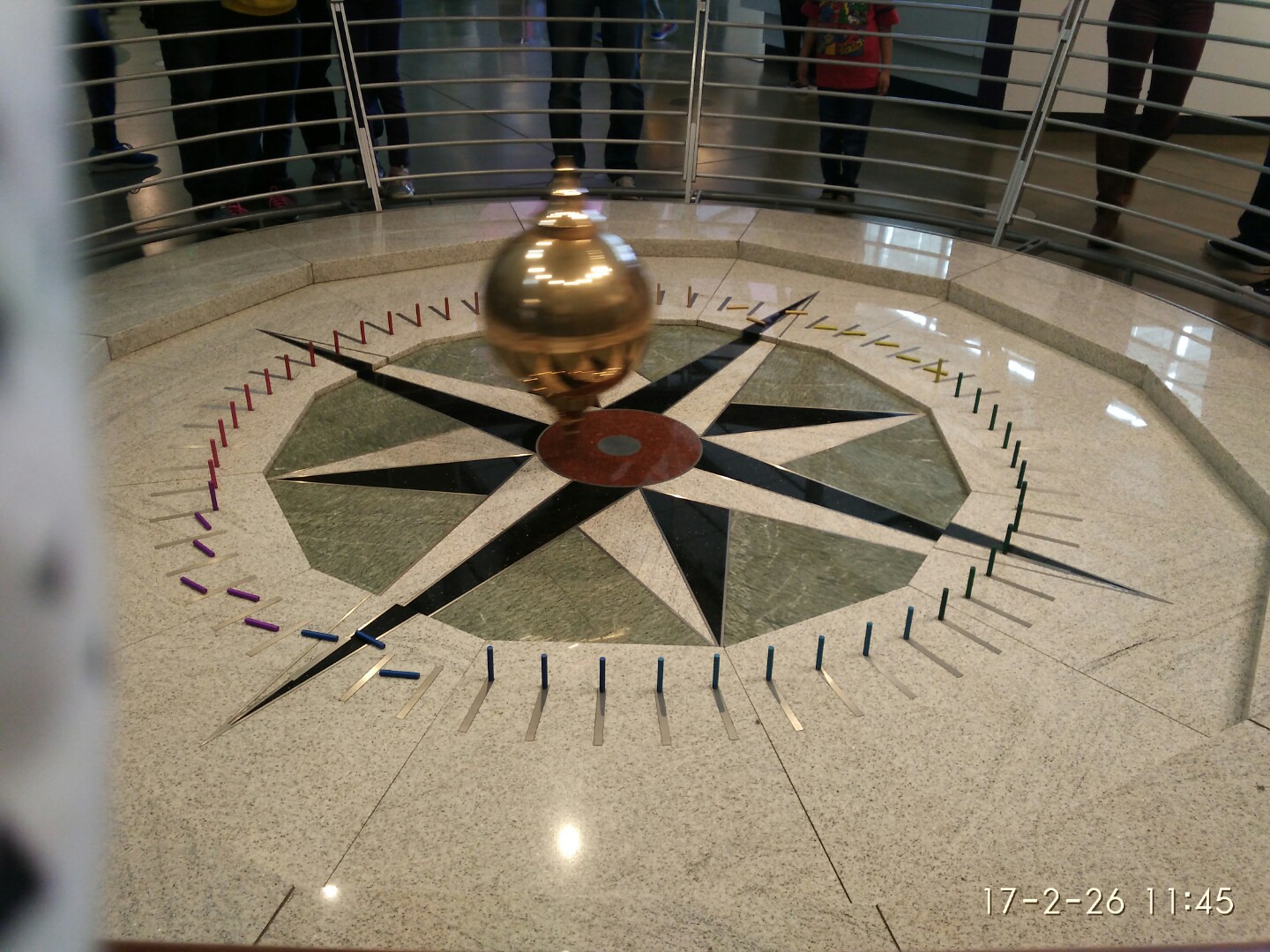The image depicts a museum installation featuring a large, marble-tiled floor with a central star pattern composed of black and white compass points directed towards each of the cardinal and intercardinal directions (north, northeast, east, southeast, south, southwest, west, northwest). At the center of this compass design sits a sizable golden ball that appears to be either suspended as part of a pendulum or spinning like a top. Surrounding this central structure are several upright pins, resembling the look of a sundial or a game of chance resembling a prize wheel. Encircling the entire setup is a gray barrier with vertical posts connected by horizontal lines, providing some level of protection yet allowing clear visibility. In the background, only the legs and waists of a group of spectators are visible as they peer over a fence at the installation, highlighting the exhibit's considerable size. The ground is a hard, smooth, shiny surface, and the scene is captured by what appears to be a security camera, as indicated by a timestamp displayed in the bottom right corner reading "17-2-26 11:45." The lighting and lack of additional text suggest a clean and focused presentation of the intriguing display.